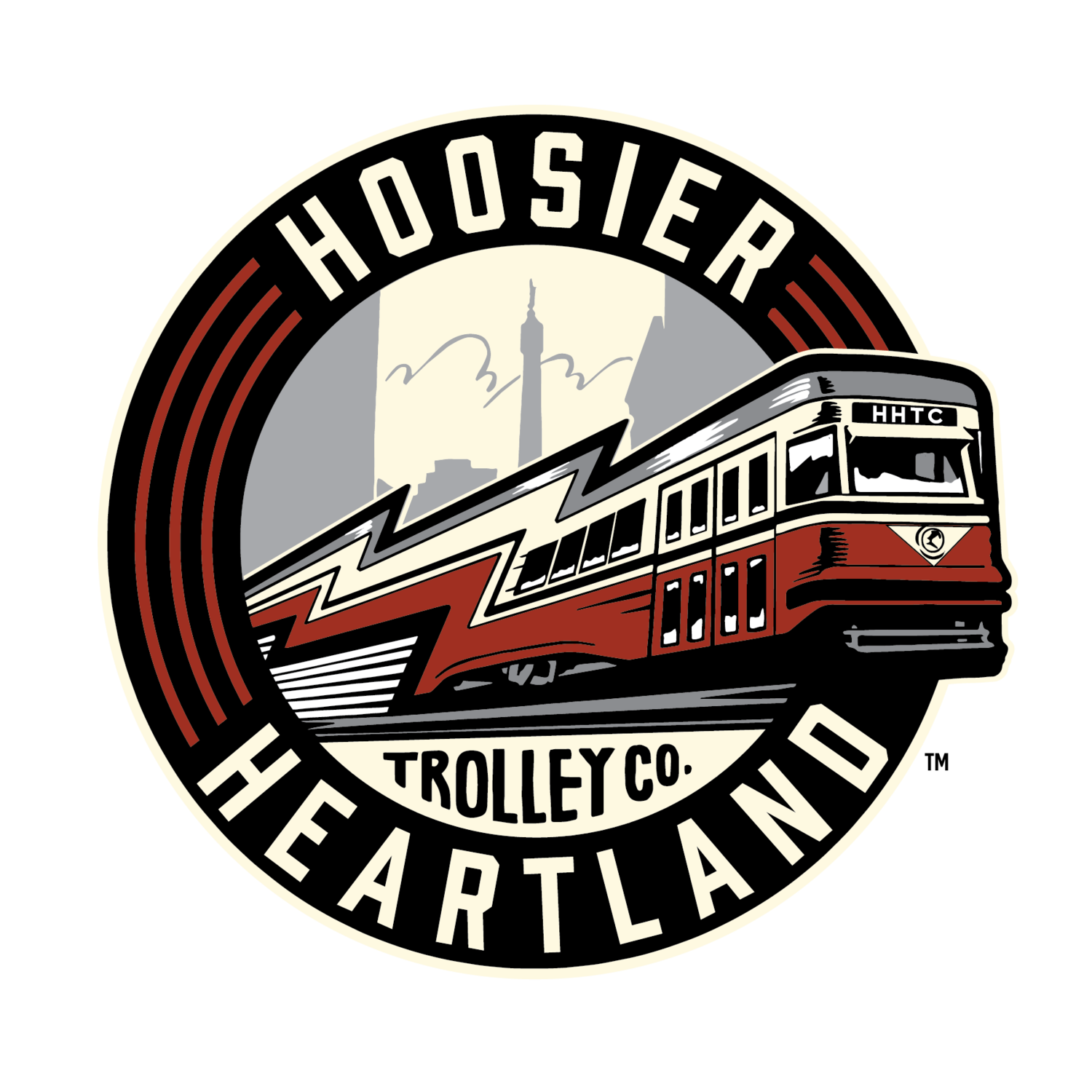The logo for the trademarked Hoosier Heartland Trolley Company is a detailed, circular emblem designed for impact. Encased within a black circle, the name of the business is prominently displayed in curved, white capital letters: "Hoosier" arches across the top, while "Heartland" mirrors it at the bottom. These are connected by three distinctive red lines running along the sides, giving a sense of coherence and motion. The centerpiece of the logo is a dynamic cityscape background, outlined in gray, against which a train appears to burst through the circle in a striking 3D effect, traveling from left to right. The train itself features a unique lightning bolt shape at its rear, signifying speed, with a red base, gray roof, and yellow windows, accented with white shading to emphasize rapid movement. Below the train, above the word "Heartland," the words "Trolley Co." are inscribed, completing the circle's intricate design. The front of the train is marked with "HHTC," encapsulating the essence of the Hoosier Heartland Trolley Company.